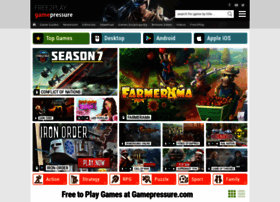The website homepage features an array of free-to-play games prominently displayed against a vibrant orange background. At the forefront, a farmer is depicted carrying a wheelbarrow, adding a rustic charm to the scene. "GamePressure.com" is written boldly, emphasizing the vast assortment of games available. Titles such as "Top Games," "Season 7," "Iron Order," and "YMA" catch the eye, each with distinctive visuals — for instance, "Iron Order" showcases an imposing gray metal tank. The interface supports multiple platforms, including desktop, Android, and Apple iOS. A search bar is positioned in the top right corner, ready to assist in navigation, while other text elements remain slightly blurred, giving a dynamic feel to the site.